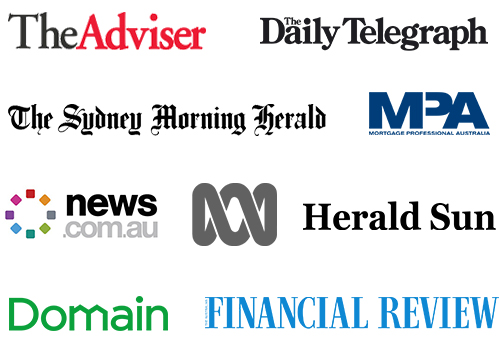A screenshot captures the display of a laptop screen showcasing a web page under the category "websites and screenshots." The web page prominently exhibits an array of eight different logos from various global publications and news sites, organized neatly into four rows with two logos in each row. These logos represent the following entities, in order: 

1. First Row: 
   - The Advisor
   - The Daily Telegraph 

2. Second Row:
   - The Sydney Morning Herald
   - MPA (Mortgage Professional Australia)

3. Third Row:
   - news.com.au
   - The Herald Sun 

4. Fourth Row:
   - Domain 
   - The Financial Review 

The combination of these logos suggests a mix of Australian and UK publications, spotlighting a global perspective but with a strong emphasis on Australian media outlets, as inferred from recognizable names like news.com.au and Mortgage Professional Australia.